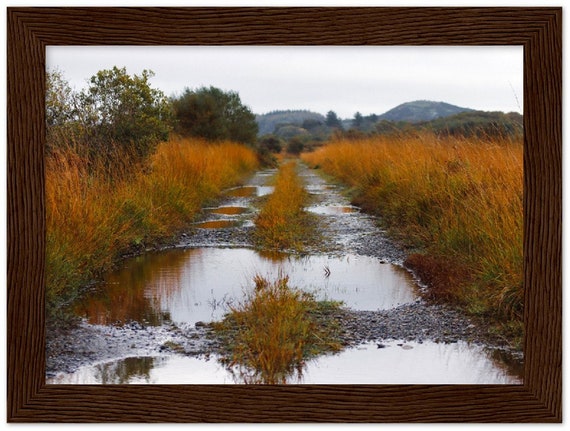The image depicts a framed photograph showcasing a desolate, abandoned gravel roadway stretching into the horizon. Encased in a rustic brown, wooden frame, the photograph invites the viewer into a remote, rural setting. The road itself is dotted with numerous puddles, suggesting a recent shower, with grass—tinged with reddish and golden hues—growing prolifically on either side and down the center where vehicle tires have long ceased to tread. The scene is framed by low-lying, pleasant trees and distant hills, often mistaken for mountains. The roadway appears lonely and unused, set in what might be a cold, rocky region such as rural Alaska or Russia, characterized by minimal vegetation. The surroundings are rich in earth tones, primarily shades of orange, green, brown, and gray, creating a harmonious, autumnal palette. The photograph captures a moment of serene abandonment, with the puddles reflecting the sky and the untouched wild grasses accentuating the solitude of the landscape.